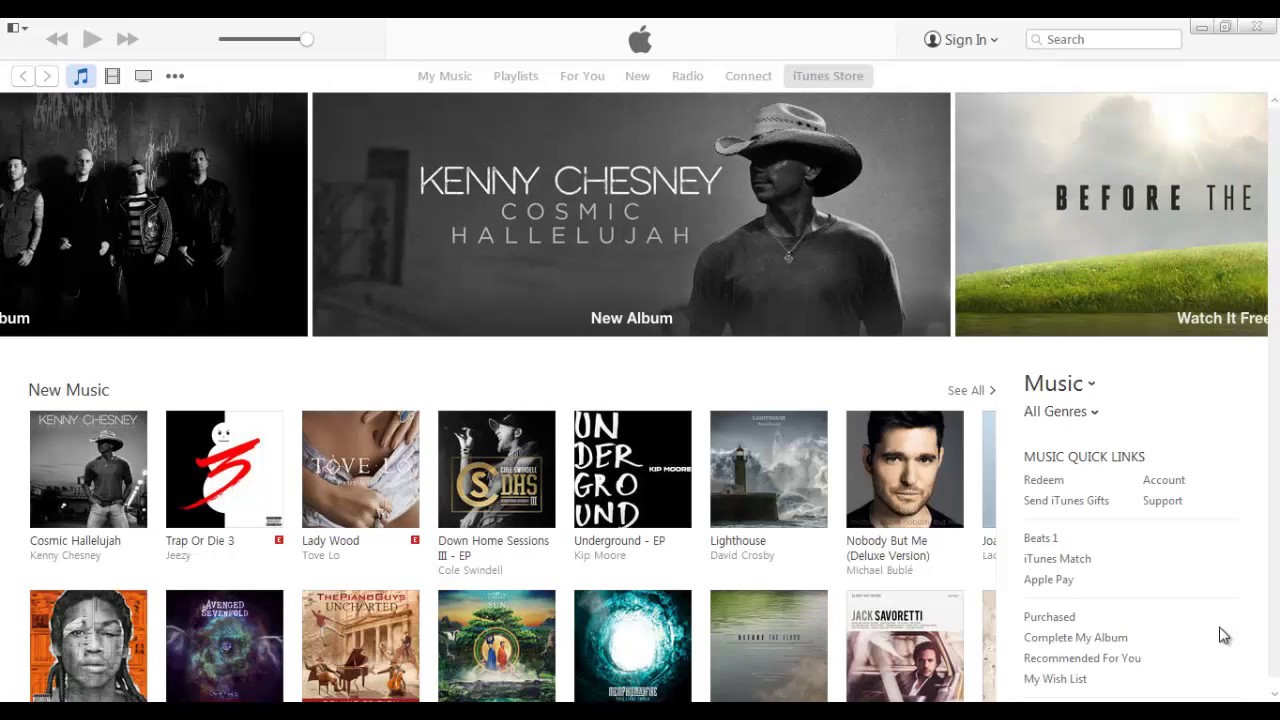This is a detailed screenshot from the Apple Music section of iTunes. The top left features standard control icons: a back arrow, play button, and forward arrow. Centered at the top is the distinctive black Apple logo with a bite taken out of the right side. On the far right of the top bar, there is a "Sign In" prompt accompanied by a search bar.

Beneath the Apple logo, there is a navigation menu listing: "My Music," "Playlists," "For You," "New," "Radio," "Connect," and "iTunes Store," with "iTunes Store" currently selected. On the left side of the main section, a partial black and white photo of a band is visible. Dominating the center is a black and white image of Kenny Chesney, a country singer. He appears to be looking to the left and is wearing a cowboy hat. The text beside his image reads: "Kenny Chesney, Cosmic Hallelujah, New Album."

To the right of Chesney's image, there is a photograph featuring a green grassy area under a cloudy sky with sunlight peeking through. The visible text reads: "Before The" with the remainder of the title cut off by the edge of the image. Below this, a list appears under the heading "New Music," which includes:

- "Cosmic Hallelujah" by Kenny Chesney
- "Trap or Die 3" by Cheesy
- "Lady Wood" by Tove Lo
- "Down Home Sessions 3 EP" by Cole Swindell
- "Underground EP" by Kip Moore
- "Lighthouse" by David Crosby
- "Nobody But Me (Deluxe Version)" by Michael Bublé

Another row of artists is partly visible but cut off at the bottom of the screen.

On the far right side, a secondary navigation menu lists: "Music," "All Genres," "Music Quick Links," "Redeem," "Account," "Send iTunes Gifts," "Support," "Beats 1," "iTunes Match," "Apple Pay," "Purchased," "Complete My Album," "Recommended For You," and "My Wishlist."